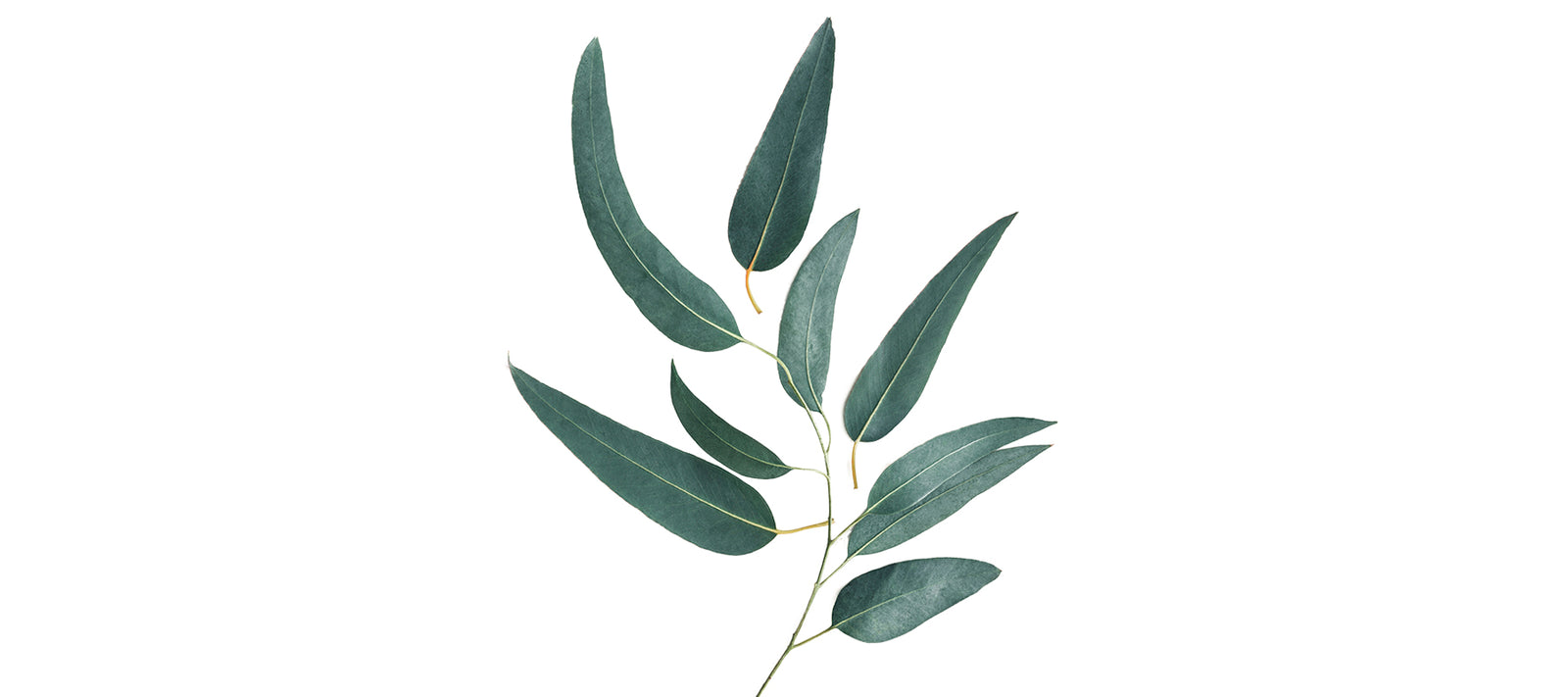The image features a thin, s-shaped branch with approximately ten oval-shaped, dark green leaves, some of which appear to have a white, powdery coating. The branch starts from the bottom, curves to the right, and then arcs back up to the left. At the top left of the branch is a prominent long, thin leaf, with a shorter leaf on the top right. Midway on the left side of the branch, there's a small leaf jutting out, and below it a larger leaf extends to the left. To the right of this large leaf, two more green leaves extend to the right, with a shorter, wider leaf situated below them. In addition, there are two unattached leaves: one long and thin with a yellowish-brown short stem at the top right of the branch, and another similar leaf below and to the right of it. The background of the photo is a simple, unobtrusive backdrop filled with clusters of green leaves.